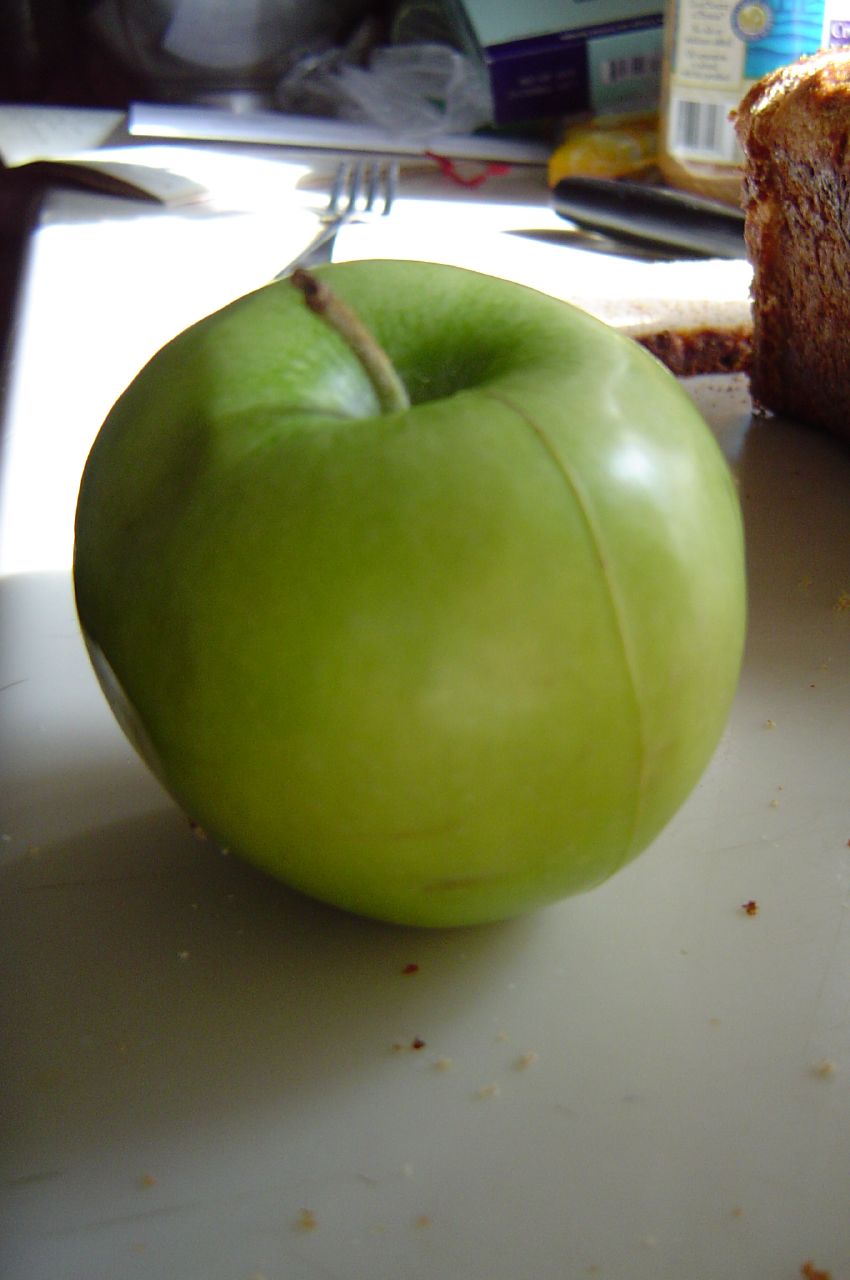The photograph captures a moment on a kitchen counter, framed by various items that tell a story of recent activity. Dominating the scene is a fresh green apple, prominently placed at the center of the white countertop. A small stem juts out from the middle of the apple, adding a touch of natural texture. In front of and behind the apple, scattered crumbs indicate recent food preparation or snacking.

To the right of the apple, a whole loaf of bread sits partially sliced, with one slice conspicuously lying loose in front of it on the counter. Sunlight streams in from an unseen source, casting a subtle glow across the countertop and illuminating a silver fork placed behind the apple.

Further to the right, there sits a collection of miscellaneous items: a yellow bottle whose contents remain a mystery, and next to it, a long, dark cylindrical object. Above these objects stands a blue box adorned with lighter blue accents. A piece of crumpled plastic lies haphazardly on the countertop next to a white piece of paper or perhaps an envelope, adding to the sense of casual disarray in this well-used kitchen space.